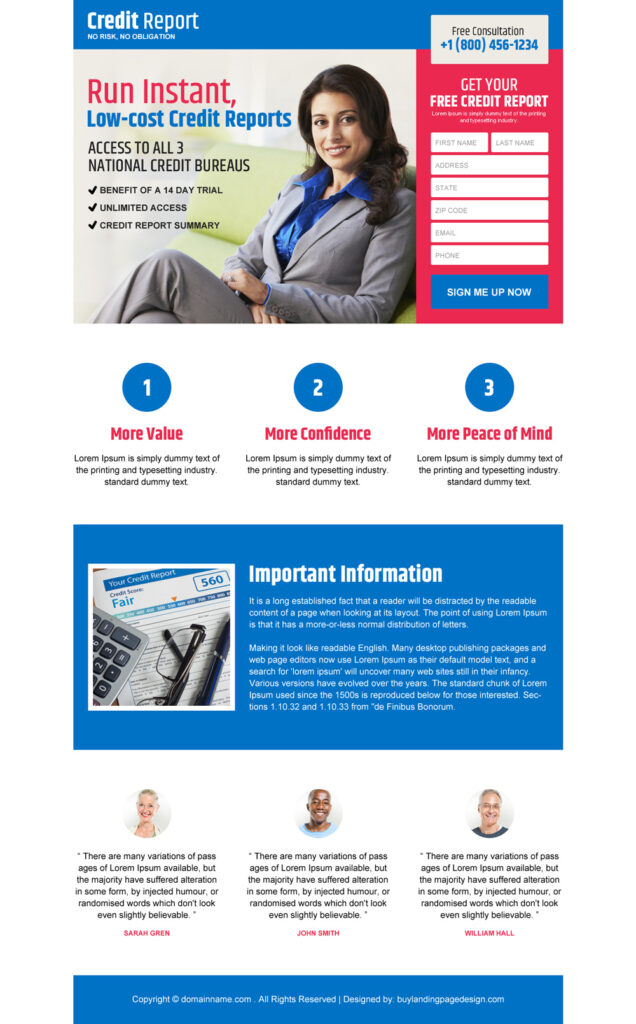The image is a detailed screenshot of a credit report website page, designed to attract users by promising a risk-free experience. On the right side, framed in a gray box, it states "Credit Report, No Risk, No Obligation." Beneath this, the offer of a "Free Consultation" is highlighted, along with a contact number: 1-800-456-1234.

Below the consultation details, the text explains the services provided, including "Instant, Low-Cost Credit Reports," with access to all three national credit bureaus. The benefits of a 14-day trial offer are described, which includes unlimited access to credit report summaries.

An image of a smiling woman in a business suit is prominently displayed, instilling a sense of professionalism and trust.

Next to the image, users are encouraged to "Get Your Free Credit Report" through a form that requires personal information: first name, last name, address, state, zip code, email, and phone number. Adjacent to the form is a bold blue button labeled "Sign Me Up Now."

Further down the page, in a white section, a simple three-step process is described with numbered entries (1, 2, 3), each paired with a brief blurb promoting "More Value," "More Confidence," and "More Peace of Mind." Accompanying these blurbs is placeholder text, indicating this part of the website might still be under development.

At the bottom of the page, there is a section titled "Important Information," which also contains placeholder text likely serving as a template awaiting final content.

The page concludes with testimonials from three individuals, though these summaries currently consist of unreadable, placeholder text, suggesting they have yet to be finalized.

Overall, the page appears to be a template for a credit report service website, prominently featuring key promotional elements and form fields essential for lead generation.